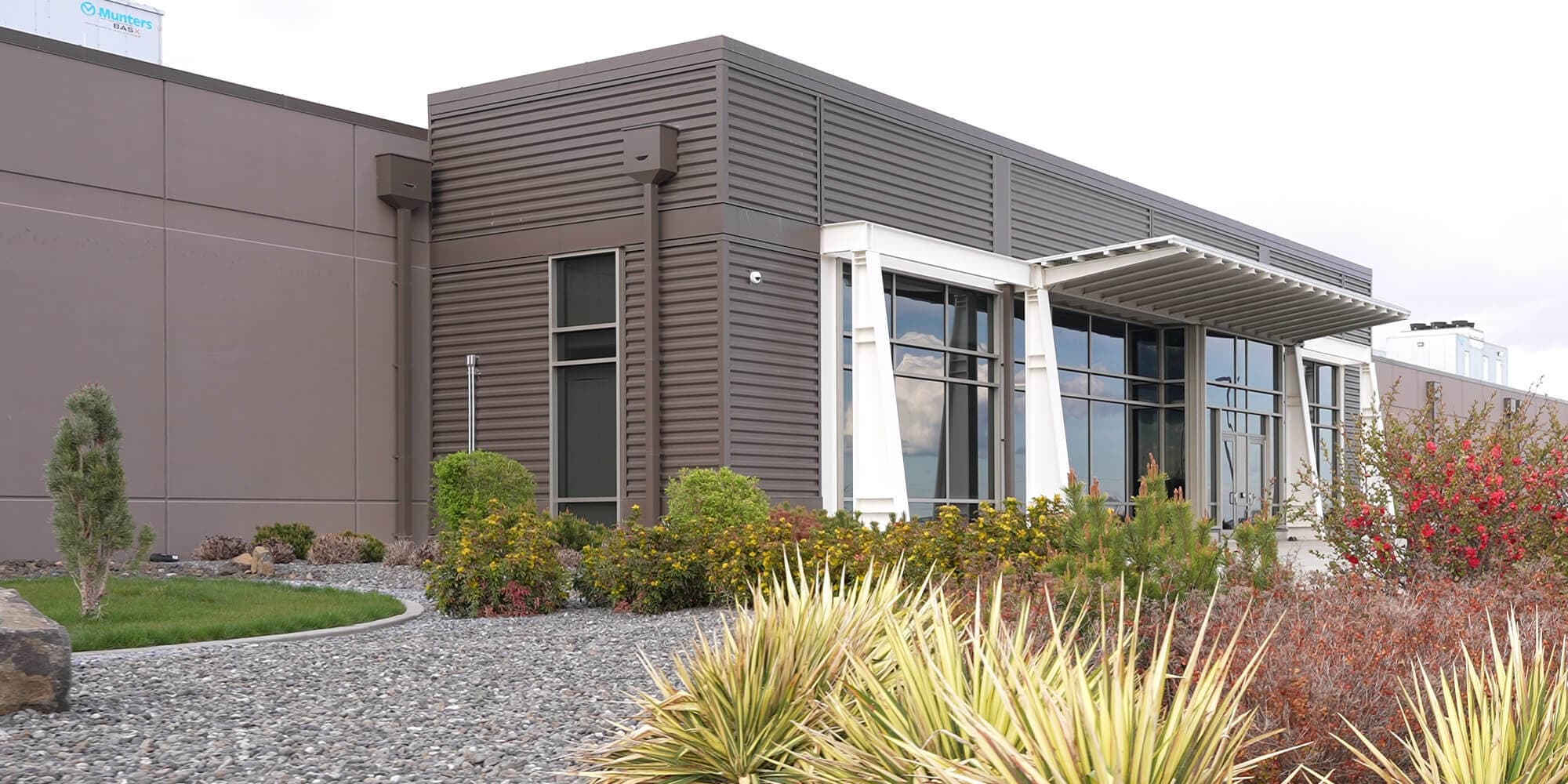This image features a single-level, brownish building that could be a house, office, or warehouse. The sky in the background is bright white, giving a cloudy appearance. The architecture includes grooved siding with a white overhang and a section of flat panels. The front facade boasts large windows and glass doors bordered with white trim or siding. Surrounding these are green and yellow plants, some resembling small aloe plants interspersed with yellow flowers. Bushes with red flowers, likely bougainvilleas, also adorn the front. A rounded grassy area with a small tree is a focal point, bordered by a pebble stone driveway and additional bushes, some of which contain little flowers. Further in the background, tall buildings are visible, adding an urban context.